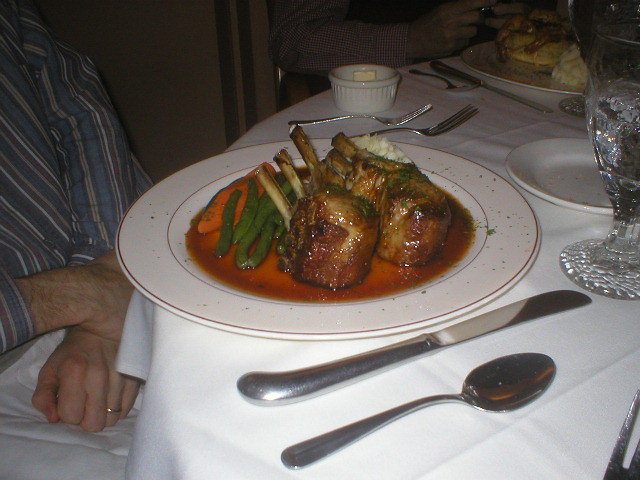The photograph captures an elegant dining scene inside a fancy restaurant featuring a round table draped with a pristine white cotton tablecloth. The main focus is on a beautifully presented plate of food. The round porcelain plate, adorned with gold rings on both the inner and outer edges, contains a lavish meal. Dominating the plate are succulent lamb shanks, bathed in a rich, reddish gravy and accompanied by a medley of green beans, carrots, and mashed potatoes. Positioned around the plate are two forks on the left, and a knife and spoon on the right. A small round butter dish and an ornate clear glass of water sit above the plate on the right, while a white bread plate remains unoccupied.

To the left of the plate, a person is seated, their posture relaxed as they lean back with their left wrist clasped in their right hand, showcasing a thin gold wedding band. They are dressed in a long-sleeved shirt featuring blue, white, and cream stripes, with a neatly placed white napkin on their lap. In the background, to the top right of the image, another diner’s plate is partially visible, hinting at the presence of an older gentleman enjoying his meal in the softly lit ambiance of the restaurant.